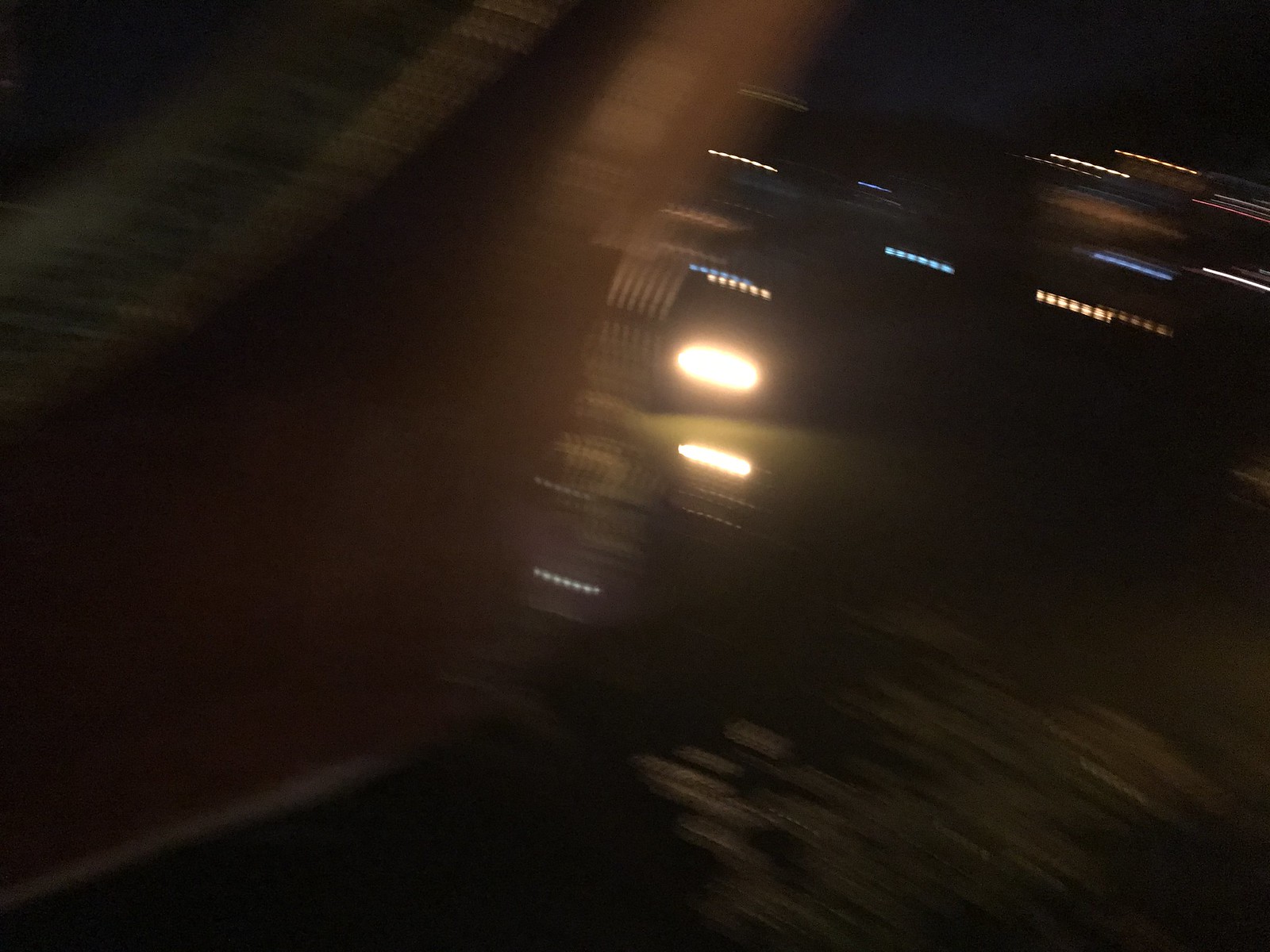This color photograph, likely taken at night, is remarkably blurry and shaky, suggesting it might have been an accidental shot. The image appears to capture a scene with two lawn lights connected to a tent, which can be vaguely discerned on the left side despite the distortion. The orientation of the photo seems off, possibly upside down or tilted, as indicated by the unusual placement of lights and what looks like tree silhouettes above them. The blur and streaks of light suggest significant movement as the picture was taken, amplifying the sense of disarray. The overall impression is of a chaotic, almost abstract image, with no clear objects or text due to the motion and poor focus.